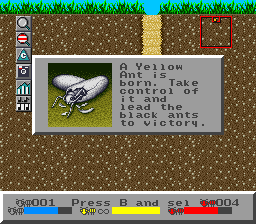The image is a screenshot from an old computer game. The central focus is a gray dialog box with text that reads, "A yellow ant is born. Take control of it and lead the black ants to victory." To the left of this text, a white egg with a white insect emerging can be seen. The background behind the dialog box depicts an underground environment with a simple design, showing brownish soil flecked with various colors. At the top of the image, green grass and a blue sky are visible. In the upper right-hand corner, there is a highlighted section of the underground game board within a black box, containing a smaller red box. Various controls and gauges are displayed at the bottom of the screen, including horizontal bars of yellow, red, and blue which likely indicate the progress or status of different players or elements within the game. Additionally, a series of square icons are seen vertically aligned in the upper left corner, and there is a horizontal gray band with black text and colored rectangles (blue, yellow, and red) near the bottom.